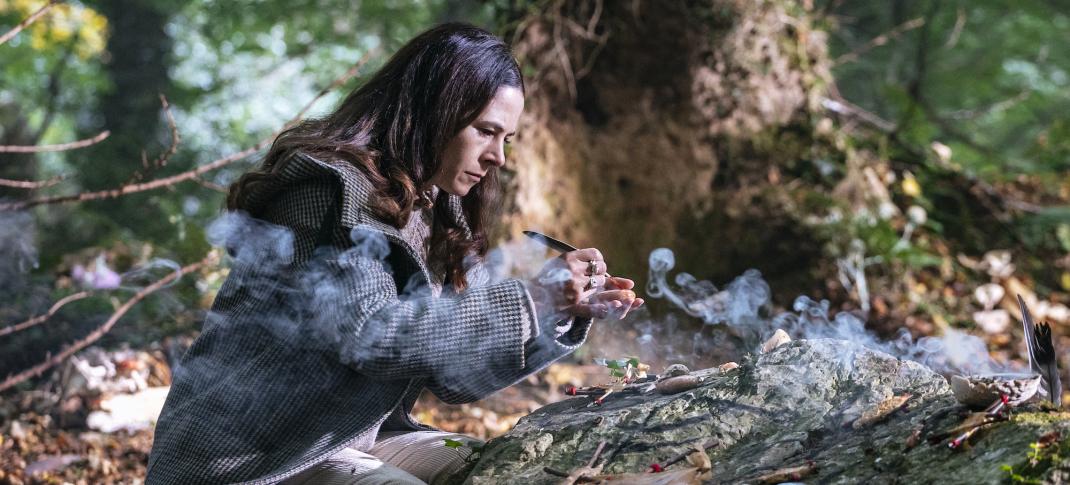This rectangular, almost banner-like photograph captures a serene moment in a forest setting, where a deeply focused woman, clad in white pants and a black-and-white checkered jacket with long sleeves, kneels in front of a large, gray dirt mound. She has long brown hair and is looking towards the bottom right, concentrating intently on an item in her hands. The item appears to be a stick that is expelling smoke. Before her, various rocks and plants are strewn around, and a small round bowl of incense emits a wispy trail of smoke. These elements, along with the presence of feathers around the mound, suggest a ceremonial or religious ritual. The background, though slightly out of focus, reveals large trees, leaves, and sunlight dappling the ground, emphasizing the natural and tranquil ambiance of the forest.